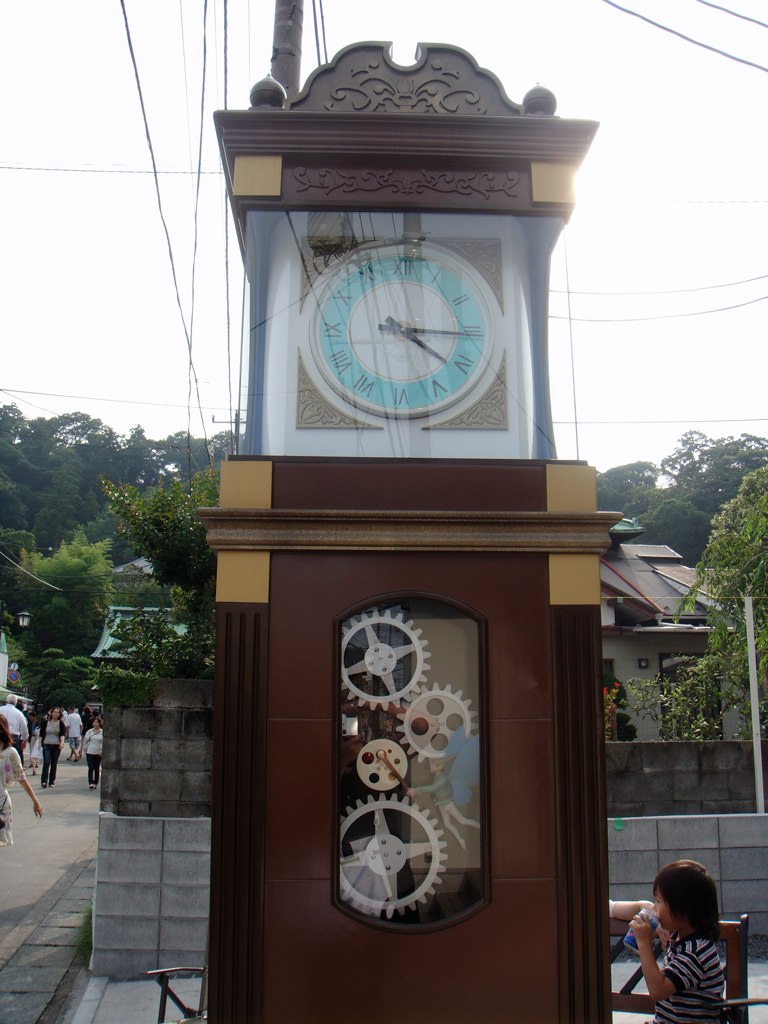In this bustling neighborhood scene, the sky is an almost pure white, casting a soft, diffused light over the area. A network of electrical lines and poles crisscrosses the view, adding a web of urban infrastructure. The roofs of several buildings peek into the frame, bordered by a sturdy concrete fence. The street below is animated with numerous people, suggesting a lively community. In the background, a line of trees provides a leafy contrast to the built environment.

Dominating the foreground, a person stands close to a prominent wooden clock. This impressive timepiece features a large glass window at its base, through which intricate cogs and gears can be seen in constant motion, revealing the clock's inner workings. The clock face itself is mounted on a square panel with a white border, enclosing a blue circle at its center. Surrounding the blue circle, black Roman numerals mark the hours, set against a white backdrop. Sharp black hands extend from the clock's center, indicating the time. Atop this elaborate mechanism rests a brown wooden cap, completing the clock's dignified appearance.